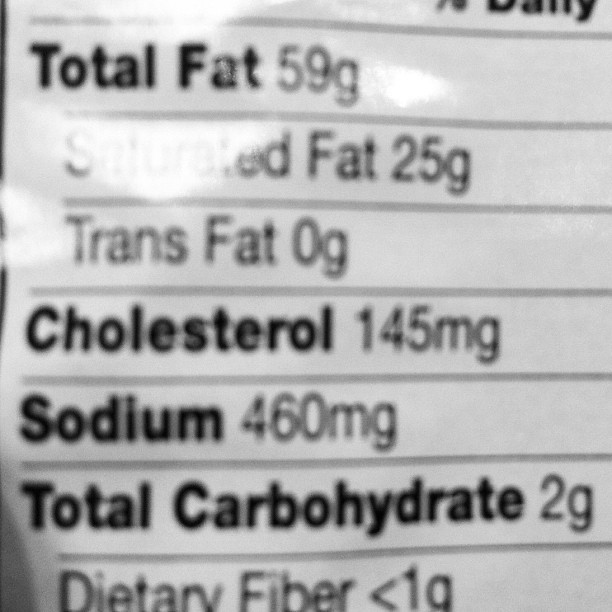A black and white photograph captures a close-up of the nutrition facts label on a food package. The label reveals the following nutritional information: total fat content is 59 grams, of which 25 grams are saturated fat, and 0 grams are trans fat. The cholesterol content is listed as 145 milligrams, and sodium is indicated at 460 milligrams. The total carbohydrate content stands at 2 grams, with dietary fiber being less than 1 gram. The image provides a clear and detailed view of these specific nutritional details, allowing for an insightful understanding of the food item's composition.